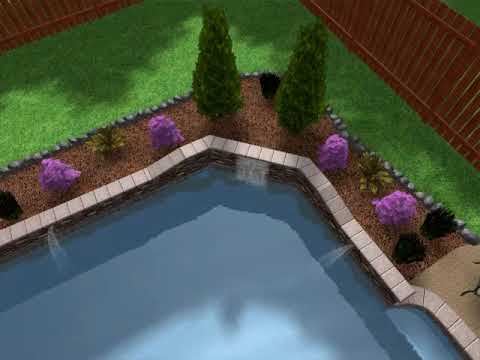The image appears to depict a blurry 3D rendering, likely from a video game like The Sims, showcasing a backyard scene. Dominating the foreground is a pool filled with bright, plastic blue water and two green lounge chairs partially submerged in the shallow end. At the top or bottom left corner lies a smaller, circular hot tub, its water contrastingly half white on the bottom and dark blue on top. Near the hot tub, there's a large umbrella with alternating white and red stripes, providing shade to a chair beside it. Below this arrangement, towards the center and bottom right, there's a landscaped garden featuring black flowers flanking both ends, leading into a patterned array of purple and green shrubs, and two trees at the far end.

In the background, a blocky house with brick-red walls and a green roof stands, featuring a wooden patio on the right side. This patio is fitted with a small barbecue area, a dining table, and chairs, adjoining a modest stone wall. The scene is completed with additional elements like tables with umbrellas and a fire pit area with surrounding chairs, set amidst a grassy expanse that envelops the entire backyard and patio area.